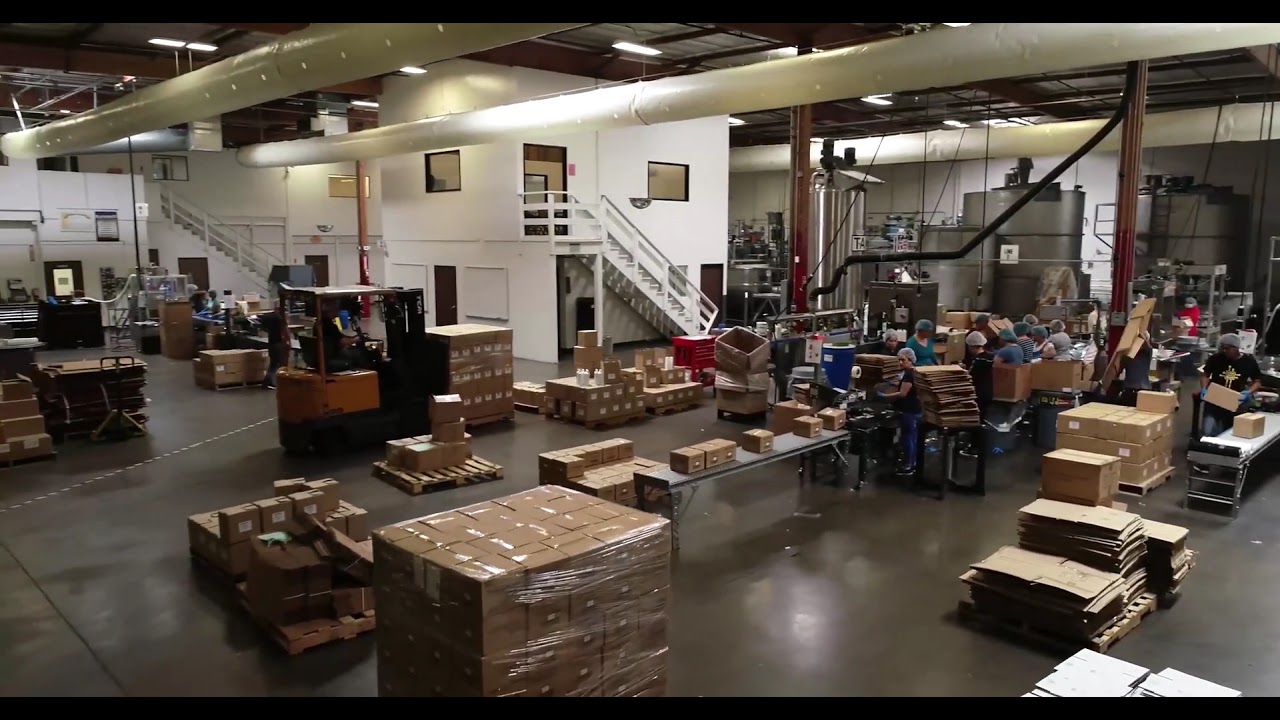The image captures the interior of a bustling factory storage area in a detailed color photograph, slightly elevated as if taken from a high vantage point or by a drone. The spacious environment features a brown concrete floor, evenly flat and clean. Central to the scene is an assembly line where workers in hairnets are busily packaging items into brown cardboard boxes, some of which are shrink-wrapped and ready for shipping. Vehicles frequently transport these boxes across the factory floor. In the background, a notable white, two-story office structure with exterior stairs ascends to a doorway on the first floor. This mid-section of the factory, framed by large white pipes running across the ceiling, connects to the brown support poles that extend from floor to ceiling. Towards the far end of the factory are large metallic containers or vats, acting as a backdrop to the clustered workers. The walls are predominantly white, harmonizing with the overhead fluorescent lighting structures. The carefully organized layout and a mix of machinery and human activity emphasize the factory’s role in production and shipment.